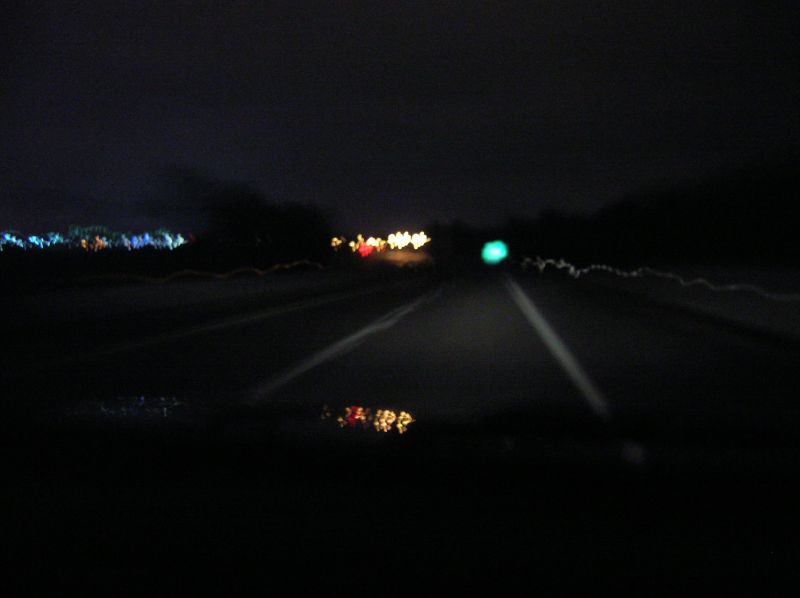A slightly blurry nighttime shot taken from inside a vehicle captures the driver's perspective of the street ahead. The scene is lit by various lights, with white lines on the asphalt clearly marking lanes. The vehicle's roof catches light glares, adding a reflective brightness to the top portion of the image. In the distance, bright lights punctuate the dark, with a distinctive reddish light standing out. To the left, blue lights mix with hints of yellow, possibly indicating a building's illumination. The overall atmosphere suggests a late-night drive through a well-lit urban area.